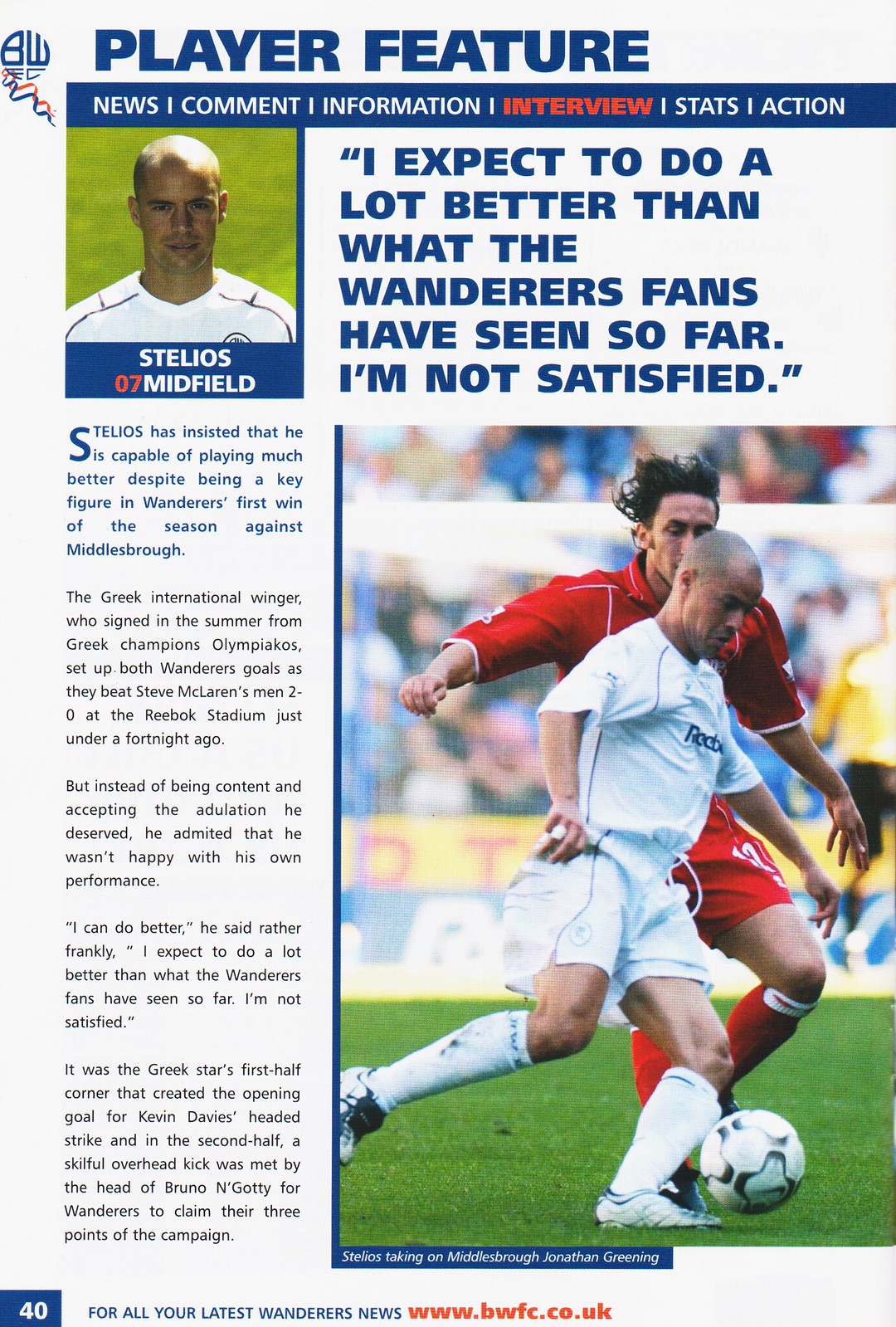The player feature from a sports magazine centers on Stelios, a Greek international winger signed from Olympiacos, who expresses his determination to improve his performance for Wanderers fans. In the article headlined with "News, Comment, Information, Interview, Stats, and Action," Stelios, positioned in midfield, is quoted saying, "I expect to do a lot better than what the Wanderers fans have seen so far. I'm not satisfied." Despite being a pivotal player in Wanderers' first victory of the season against Middlesbrough, where he assisted both goals in a 2-0 win at the Reebok Stadium, Stelios remains critical of his own play. His perfectly executed first-half corner led to Kevin Davies' headed goal, and his skillful overhead kick in the second half set up Bruno N'Gotty's header, securing three crucial points. The feature includes a headshot of Stelios and an action shot of him running with the ball, pursued by a defender in red. The article, detailed in blue and black text, emphasizes Stelios' commitment to elevate his game further, spread across page 40, with more Wanderers news available at bwfc.co.uk.